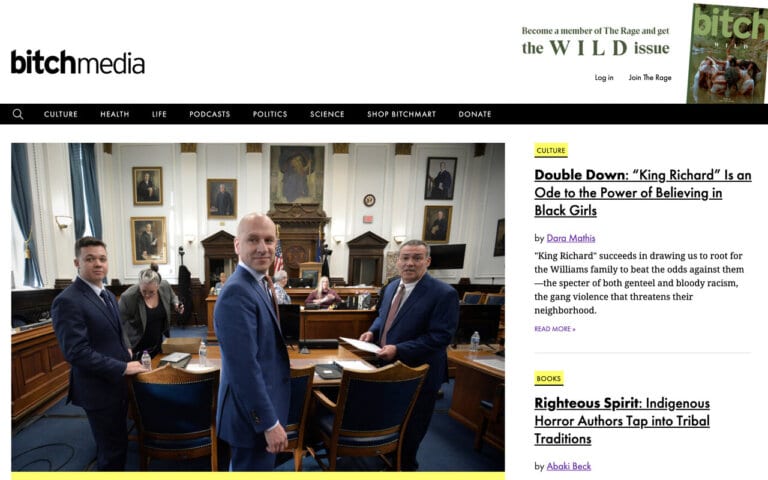This screenshot captures a segment of the Bitch Media website. In the upper left corner, the website's title, "Bitch Media," is prominently displayed. Across the top of the screen, a green banner stretches to the right side, containing the text, "Become a member of The Rage and get The Wild issue." Below this banner, an image of a magazine cover is visible, featuring the word "Bitch" in bold letters, followed by "The Wild Issue." Beneath this image, the text invites users to "Log in and join The Rage." A black bar spans the width of the page, displaying the call to action "Join The Rage" in clear, white font.